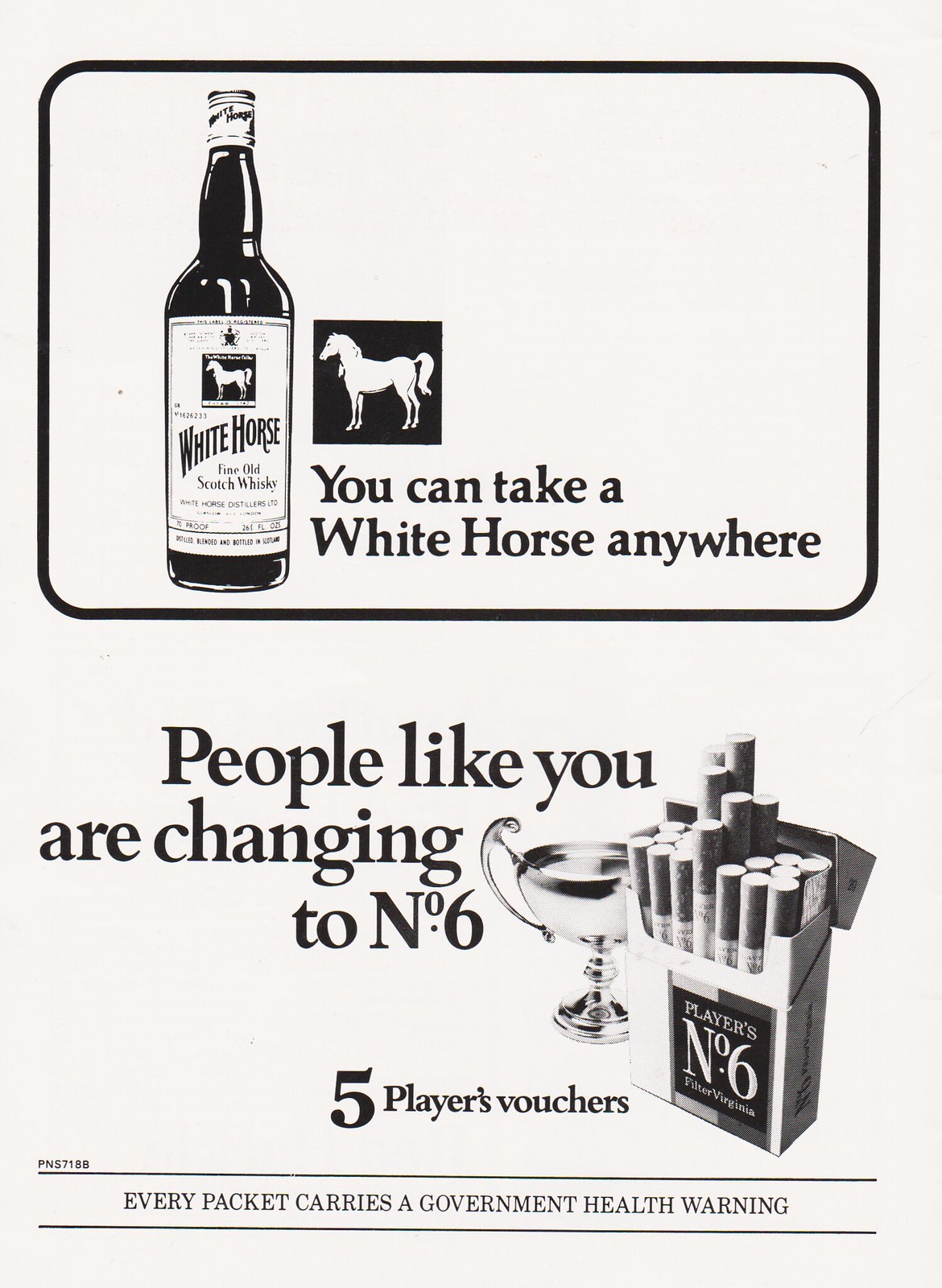The vertically aligned rectangular black-and-white image appears to be a photograph of a page from an old magazine or newspaper featuring two advertisements stacked one above the other. The top advertisement is for fine old Scotch whiskey under the brand "White Horse." Enclosed within a medium-sized black border with curved edges and a light gray background, it prominently displays a black-and-white bottle of White Horse whiskey positioned on the left. The bottle has a white label with black text that reads "WHITE HORSE" in an inclined serif font, with larger "W" and "H", and "Fine Old Scotch Whiskey" written beneath it in smaller print. Adjacent to the bottle is a small black square containing an image of a white horse, underneath which the text reads, "YOU CAN TAKE A WHITE HORSE ANYWHERE."

The bottom advertisement promotes "Players Number 6" cigarettes. It is set on a white background with no additional border details. The black text at the top states, "PEOPLE LIKE YOU ARE CHANGING TO NUMBER 6." To the right, there is a black-and-white photograph of a pack of Players Number 6 cigarettes with a few cigarettes protruding from the top, alongside what appears to be a mixed drink in a glass. Below this, the text reads "FIVE PLAYERS VOUCHERS." At the very bottom, within a demarcated area formed by a black line above and below the text, it reads, "EVERY PACKET CARRIES A GOVERNMENT HEALTH WARNING." This bottom text also appears in a serif font, maintaining consistency with the upper advertisement.